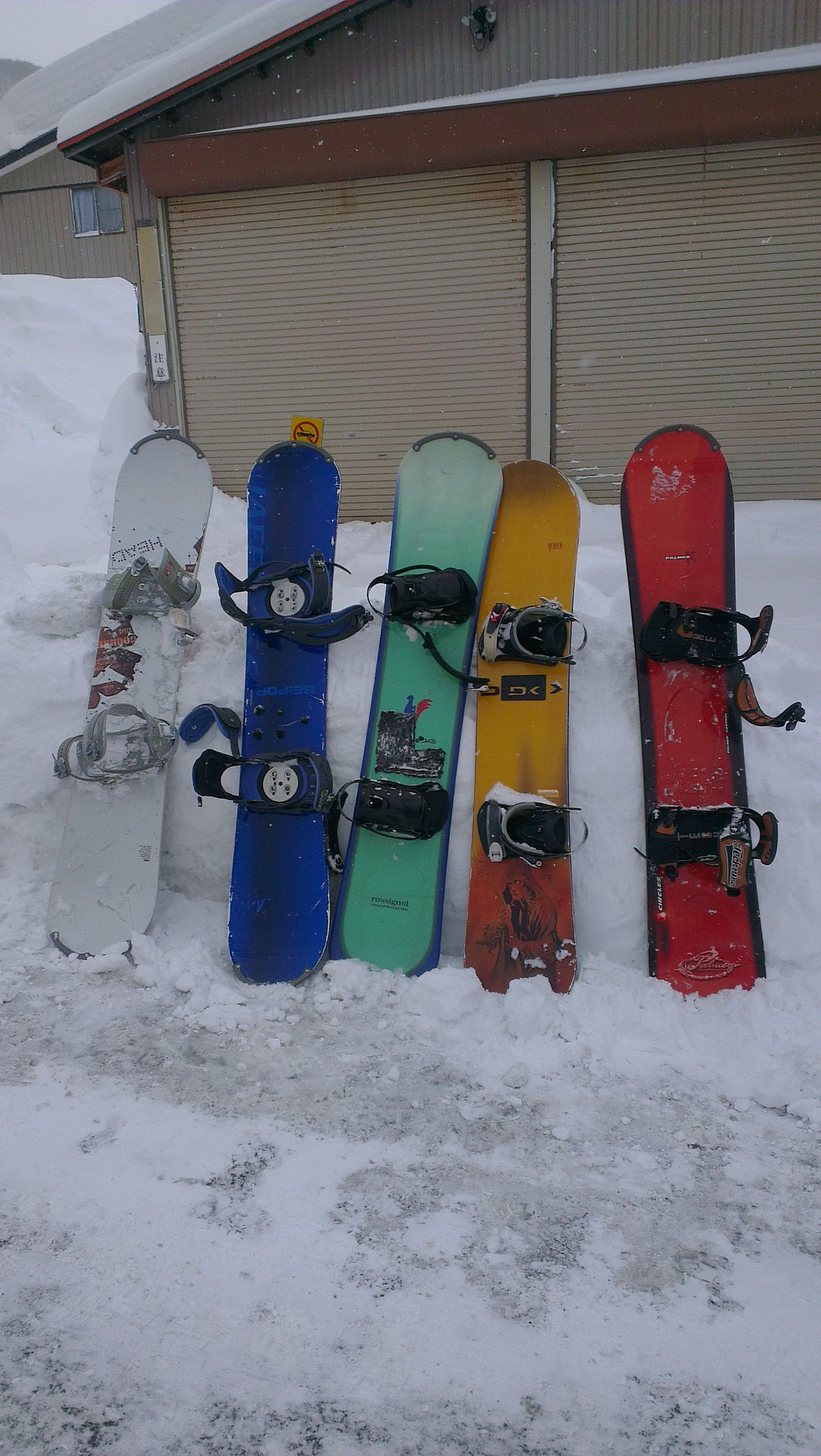This color photograph captures a detailed winter scene featuring a row of five snowboards propped against a large mound of hard-packed snow, possibly created by a snowplow. The snowboards, lined up from left to right, are predominantly white, blue, turquoise, gold, and red, each with bindings for attaching riders' feet. The bindings on the leftmost snowboard are light gray, while the rest have black bindings. The background reveals a beige metal building with two corrugated roll-up garage doors and a gable roof dusted with snow. The snow in the foreground appears dirty and grayish, suggesting a plowed paved surface, such as a parking lot or driveway. The photograph, taken in a vertical orientation, showcases the snowy scene with the colorful snowboards standing out against the wintry backdrop.